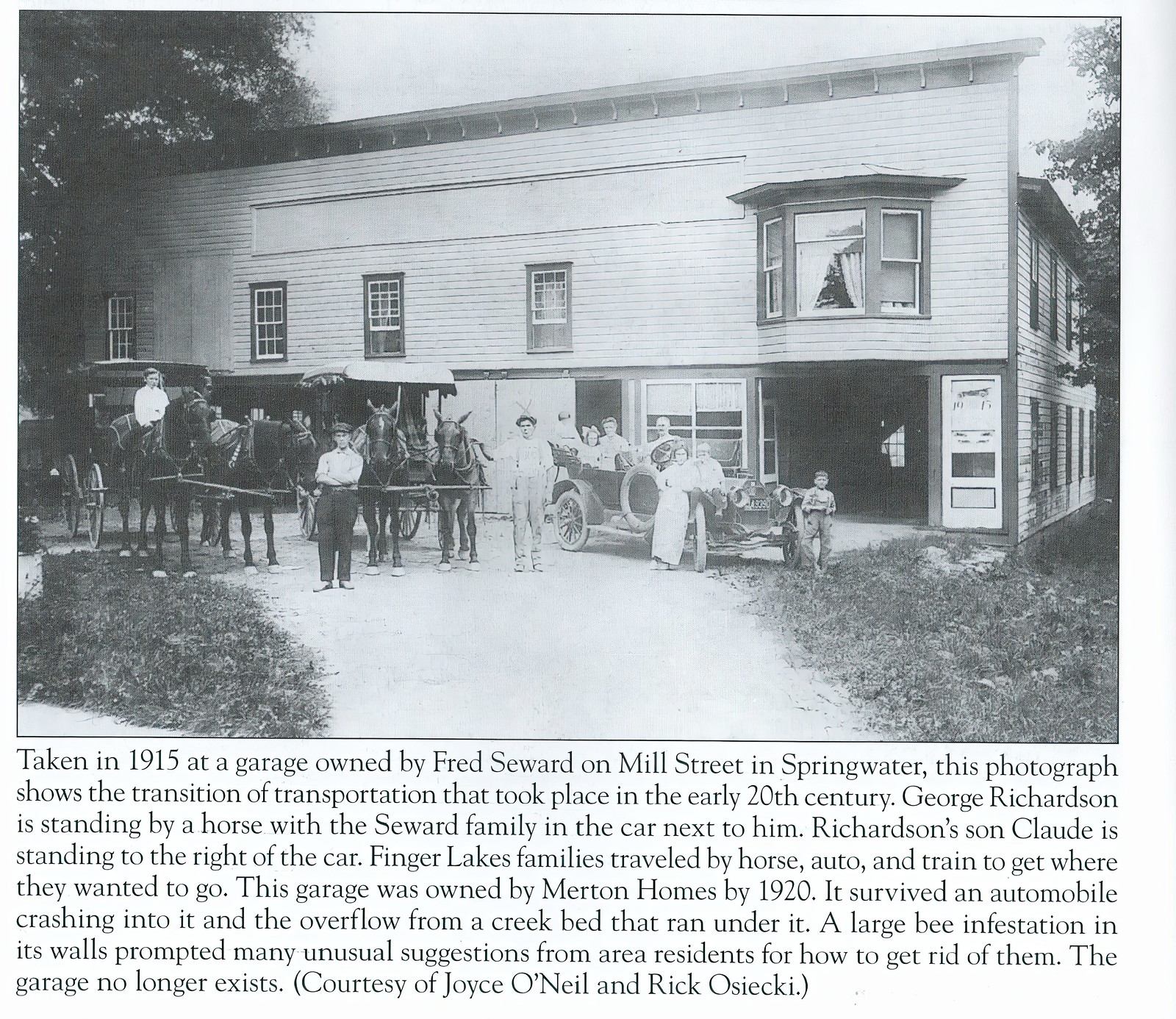This is a black and white photograph taken in 1915, depicting the transition of transportation in the early 20th century. The scene captures a two-story building in the background, identified as a garage owned by Fred Seward on Mill Street in Springwater. The upper floor features four windows on the left side and a bay window on the right, directly above a large entrance on the first floor. 

In front of this garage, a diverse group of people and modes of transportation are assembled. On the left, there is a carriage with several horses; one man is mounted on a horse, and another stands in front of them. Towards the center, a vintage open-air automobile is parked, occupied by the Seward family, with George Richardson standing by the horse next to it. His son, Claude, is positioned to the right of the car. 

The photograph, a part of a larger document with text at the bottom, evidences the era's transportation transition, featuring both horse-drawn vehicles and early automobiles. The garage, notable for Fred Seward’s ownership in 1915 and later Merton Holmes’ ownership in 1920, encountered an array of incidents including an automobile crash and a significant bee infestation. The image is courtesy of Joyce O'Neill and Rick Oseki, depicting a time when Finger Lakes families traveled by horse, auto, and train.